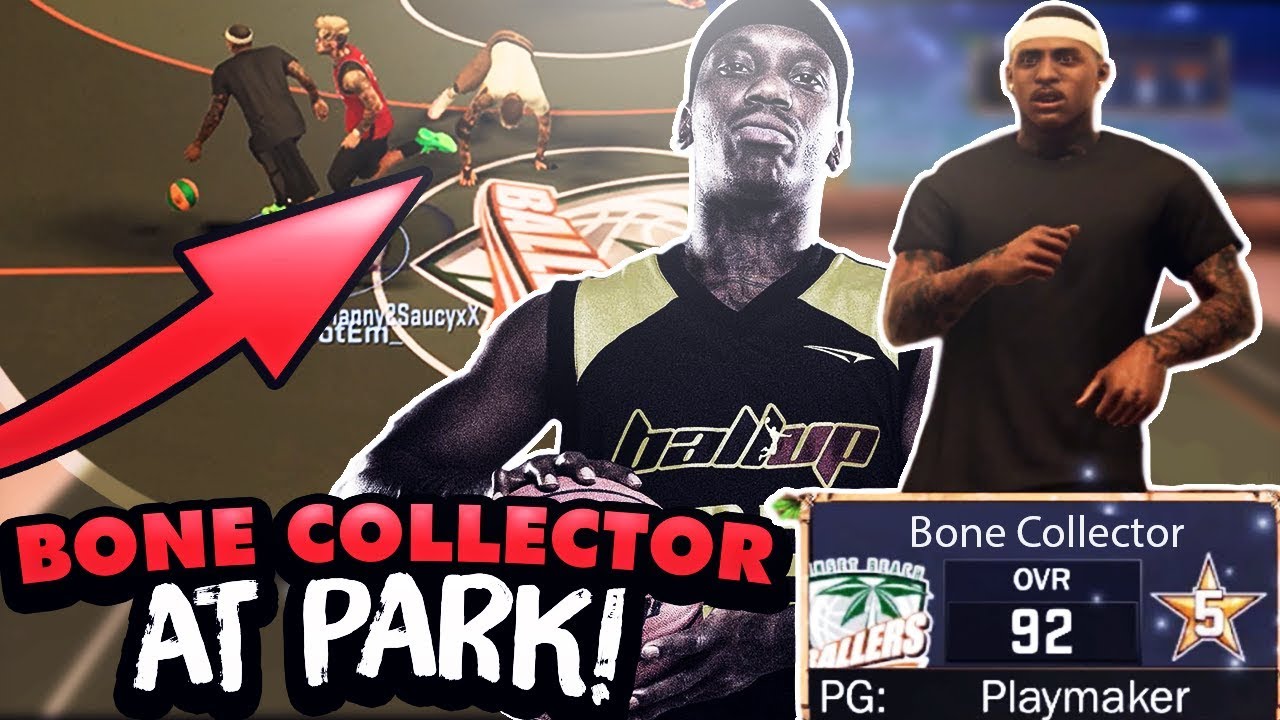The image illustrates a dynamic basketball scene set on an outdoor court. In the background, three players are deeply engaged in the game. One player, dressed in a black top and black pants, is dribbling the basketball while bent forward. Standing next to him is another player in a red tank top and black shorts, appearing to be in motion as if running. The third player, slightly back, is wearing a white t-shirt and long brown pants, also seemingly part of the fast-paced action.

A prominent red arrow, outlined in black, emerges from the bottom left corner of the image, pointing towards the text "Bone Collector at Park!" boldly written within the arrow.

Additionally, the image contains two inset graphics. The first inset shows a still of a man holding a basketball, wearing a shirt with the slogan "Ball Up." The second inset presents another man in a different setting or at a different time, dressed in a black t-shirt and a white headband, caught mid-run. This inset is labeled with the text "Bone Collector OVR 92 PG Playmaker."

Overall, the composition effectively emphasizes the intensity and skill of street basketball.